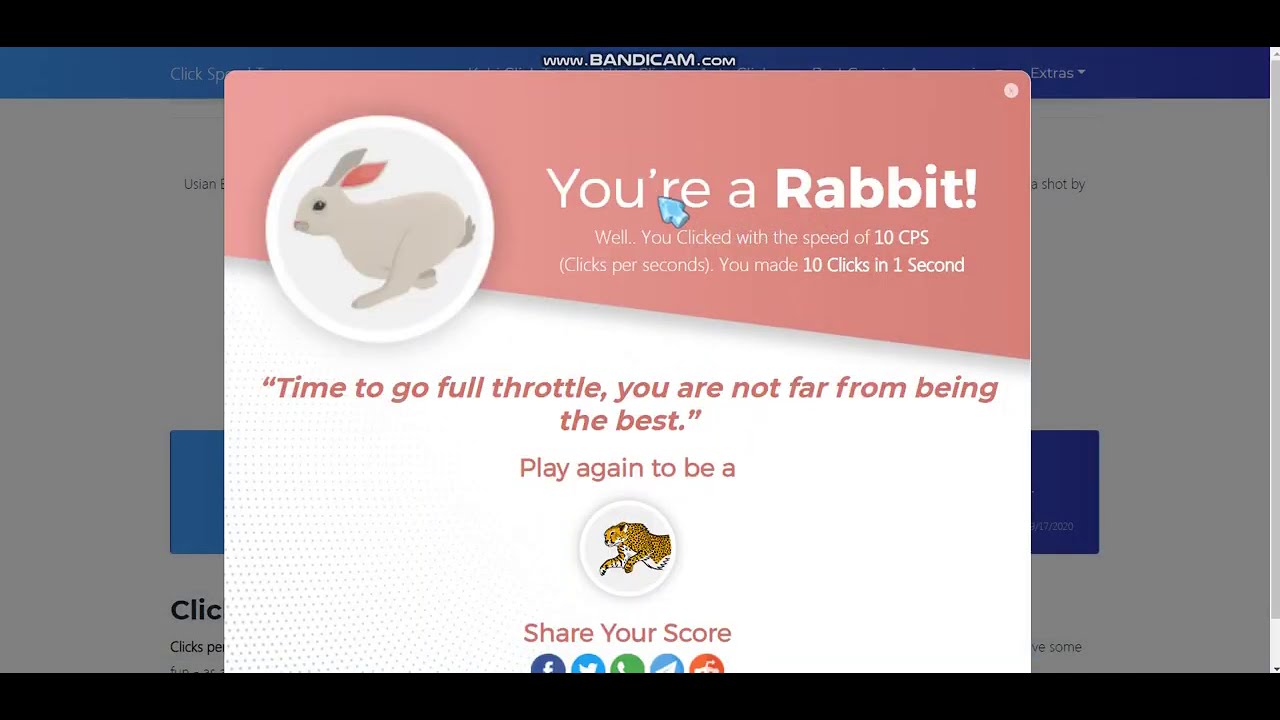The image frame is horizontally rectangular, bordered by narrow black strips on the top and bottom edges. Just below the top black border, a light blue horizontal banner spans the width of the frame. The banner contains a white text that reads "www.bandicam.com." However, the majority of this web page is obscured by a central pop-up window.

The pop-up window features a prominent image in the upper left corner: a rabbit encased in a white circle. Next to this image, text reads: "You're a rabbit. Well, you clicked with the speed of 10 CPS (clicks per second). You made 10 clicks in one second." Following this, it prompts the user with motivational text: "Time to go full throttle. You are not far from being the best."

Further down, the pop-up displays another white circle containing an image of a tiger. Beneath this, there is an invitation for users to share their achievements, accompanied by various social media icons.